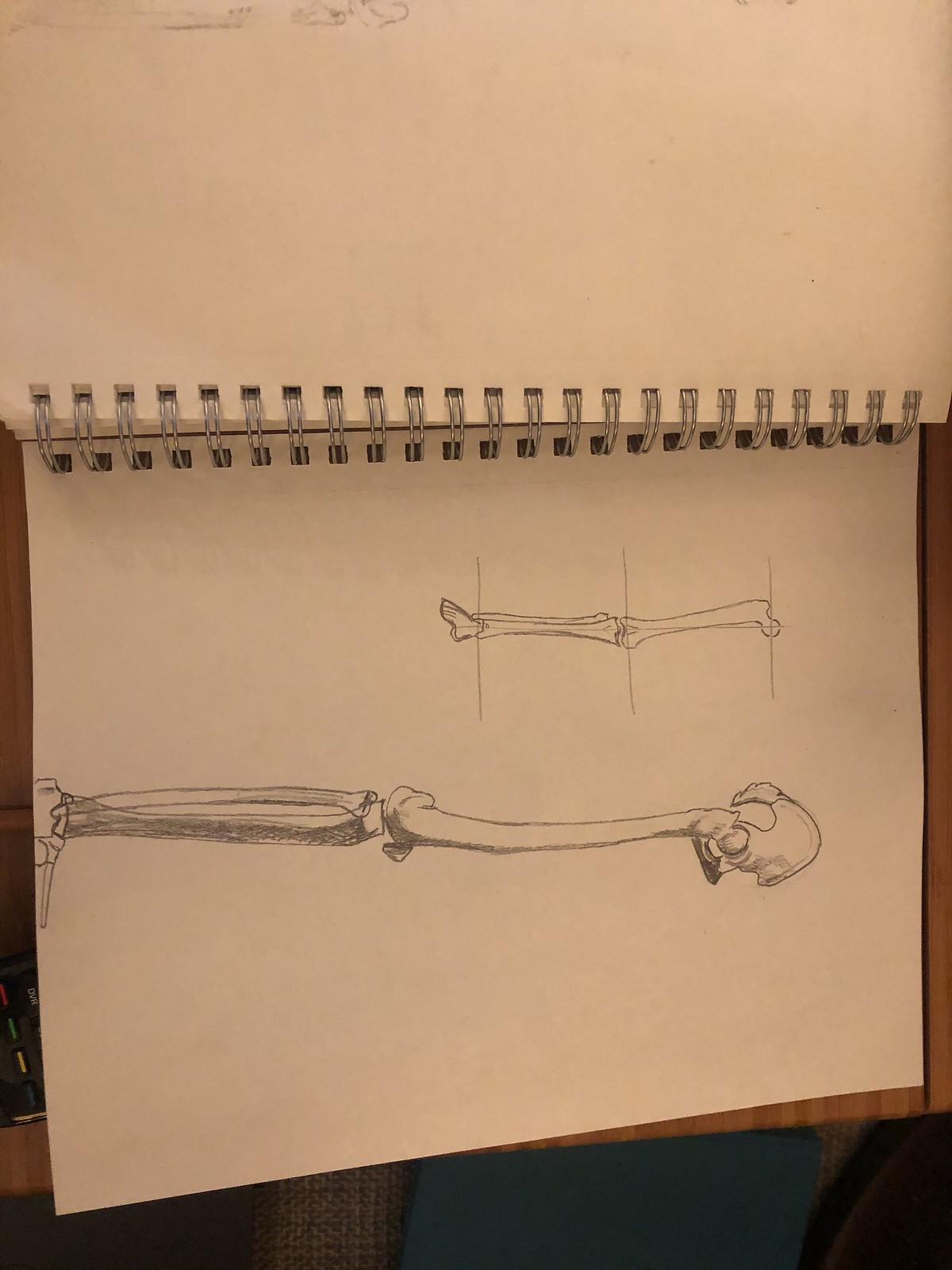This photograph captures a spiral-bound sketchbook laid sideways on a wooden table. The sketchbook, with its white pages and silver double-ringed spiral binding, is open to a detailed pencil drawing of a human leg. The larger central sketch illustrates the leg from the hip joint down to the flat-lying foot, including the femur, patella, and shin. Towards the top left of the page, there's a smaller drawing that similarly depicts the femur, marked with lines at the top, middle, and bottom to indicate different sections. The right side of the image appears darker, obscuring details on the floor beneath the table. The wooden table adds a rustic background to the intricate anatomical sketches.